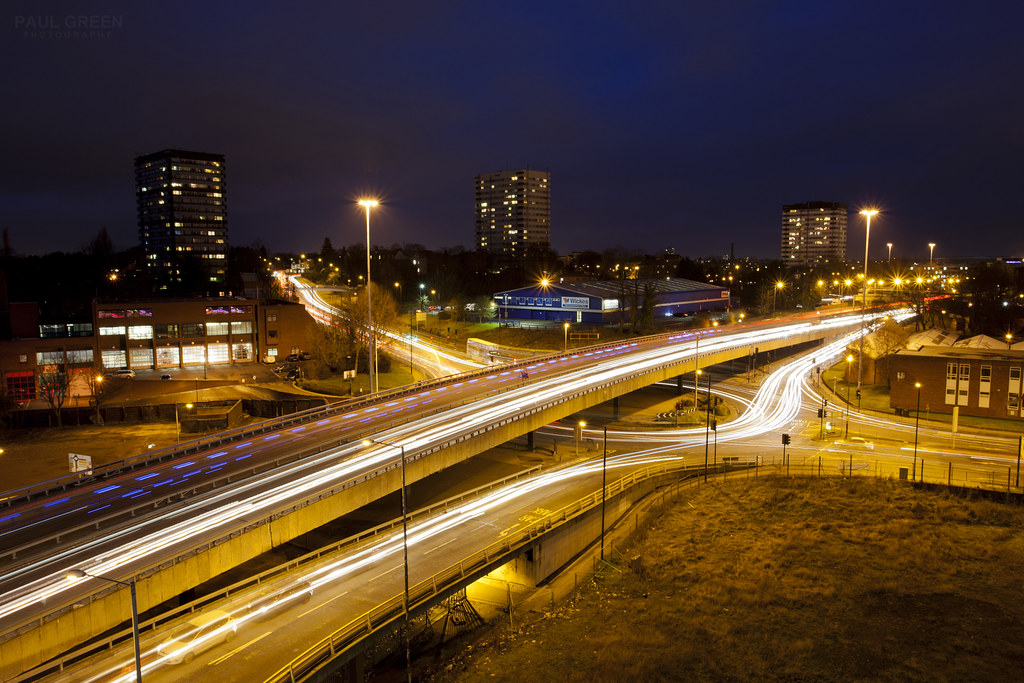This nighttime aerial photo captures a bustling cityscape centered around a freeway and its off-ramp. The main interstate runs diagonally from the bottom left to the middle right of the image, adorned with light poles on either side and dotted blue lights marking its lanes. The roundabout visible just after the off-ramp connects to a street passing beneath the highway, highlighting the intricate network of roads. The image is a time-lapse, evident from the streaks of light that reflect the movement of cars and create a dynamic flow of illuminated trails across the freeway and roundabout. In the bottom right, a grassy knoll adds a touch of green amidst the urban setting. The upper section of the photo features several tall buildings, including illuminated office towers and a blue warehouse-like structure, with streetlights casting a glow over the scene. The night sky frames this vivid urban tapestry, showcasing the city's vibrant nighttime activity.